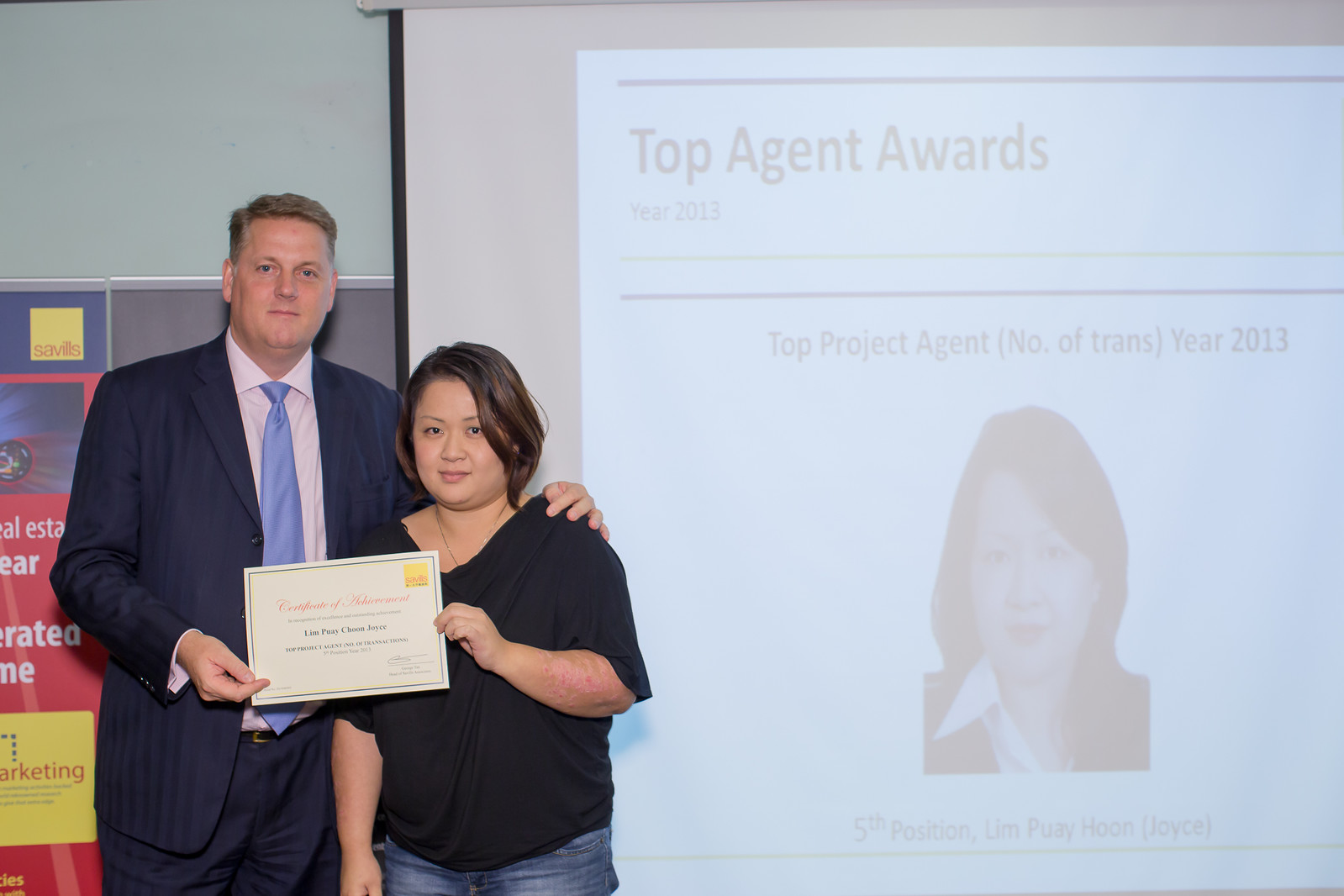This photograph captures a moment of recognition at a real estate agency's "Top Agent Awards Year 2013" ceremony. A taller man with blonde, graying hair, dressed in a blue suit with stripes, a light-colored shirt, and a light blue tie, is presenting a Certificate of Achievement to a woman named Joyce, or Mrs. Lim Pui Hoon, who is wearing a black blouse and blue jeans. The man has his hand on Joyce's left shoulder as they both hold the certificate. Behind them, a projector screen displays the award details, showing Joyce’s photo labeled "fifth position," and the text "Top Agent Awards, Year 2013," "Top Project Agent (Number of Transactions)," and "Year 2013." There is also a partially visible sign about marketing and real estate.